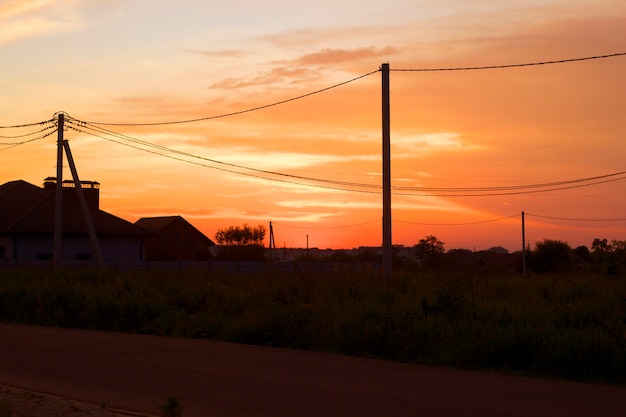This photorealistic image captures a serene sunset in a rural setting. The sky is a vivid tapestry of orange, yellow, and red hues, with tinges of blue higher up, accentuated by scattered clouds that add depth and drama to the scene. The sun hasn't quite broken through, casting a warm glow that silhouettes the landscape beneath. A prominently dark silhouette marks the land, contrasted by a network of telephone poles and power lines that traverse from the left side and continue across the right, with a central pole anchoring the composition. In the foreground, a reddish dirt road runs parallel to the scene, flanked by thick, dense green brush and wild plants. On the left side, a small house with a reddish-brown roof and possibly purple or white walls sits quietly, while further back to the right, larger trees loom. The distant roofs and silhouettes of houses blend into the meeting horizon. This peaceful yet evocative image is a perfect blend of natural beauty and rural simplicity.